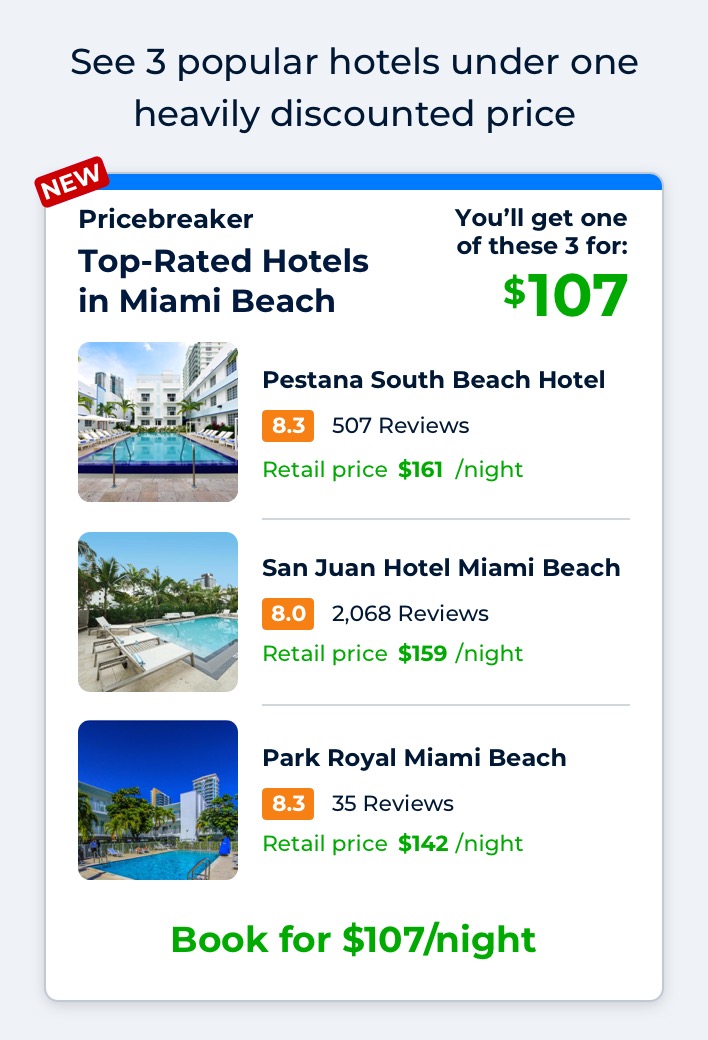The image displays an advertisement for a booking site, promoting a limited-time offer on three popular hotels in Miami Beach. At the top, bold text reads, "Three Popular Hotels Under One Heavily Discounted Price." In the top-left corner, a red and white label says "NEW." Below, a highlighted banner states, "Price Breaker: Top-Rated Hotels in Miami Beach," with a tagline to the right that reads, "You'll get one of these three for $107 per night."

The featured hotels include the following:

1. **Pistana South Beach Hotel** - Showcasing a picturesque view of its pool, this hotel boasts an 8.3 rating based on 507 reviews. The standard retail price is $161 per night.

2. **San Juan Hotel Miami Beach** - This hotel is depicted with a stunning poolside view. It typically costs $159 per night.

3. **Park Royal Miami Beach** - Illustrated with another inviting poolside scene, this hotel has an 8.3 rating from 35 reviews. The usual price is $142 per night.

The bottom of the ad prominently features the green text, "Book for $107 per night," emphasizing the special deal.